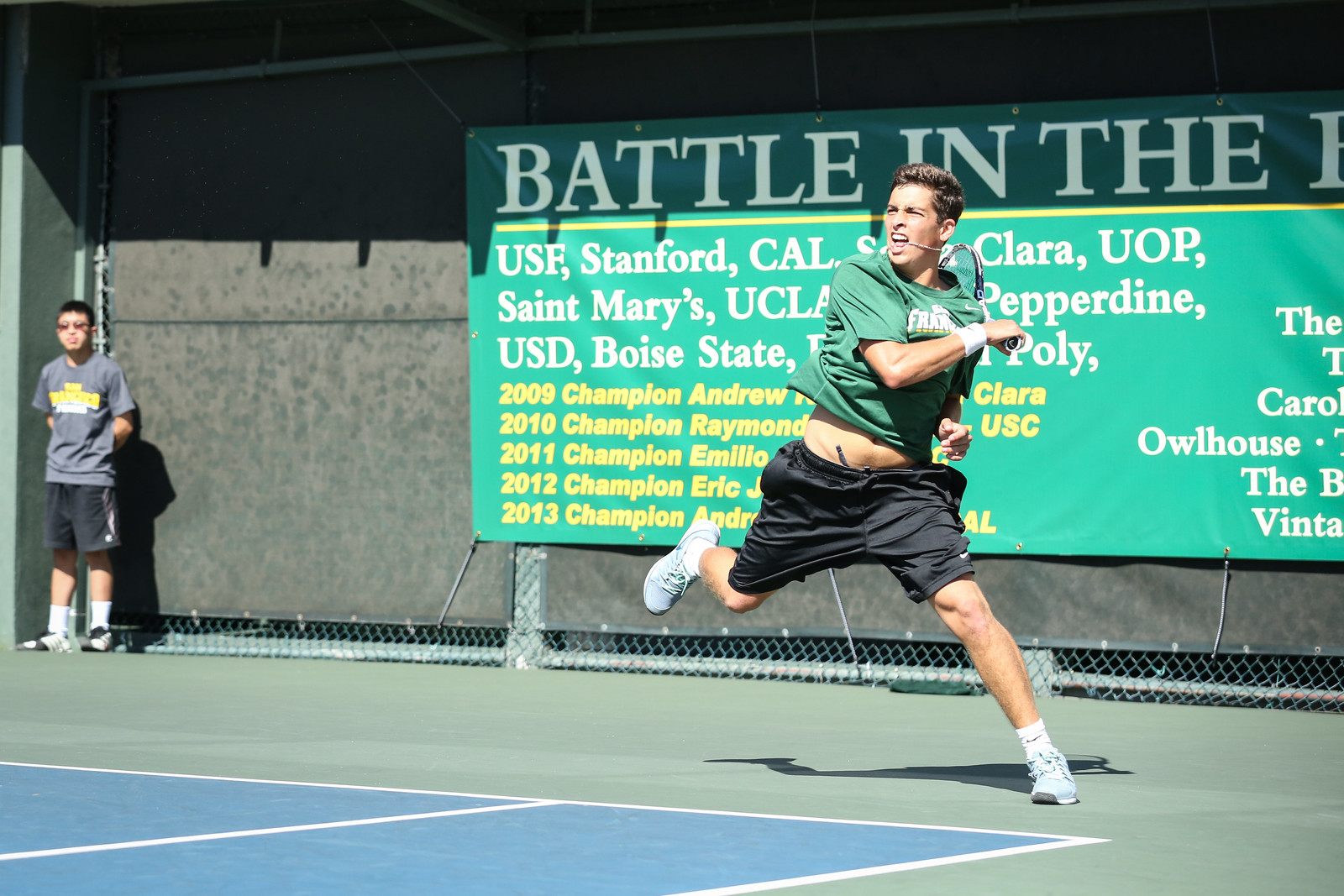This vivid photograph captures a dynamic moment during a daytime tennis match on a hard court, which features a blue playing area framed by green-out-of-bounds zones. The central figure, an overweight man in mid-swing, wears a green shirt that reveals his protruding belly, black shorts, white socks, and white sneakers. His racket is positioned across his chest, hinting at the power behind his recent hit. The background features a young ball boy wearing a gray shirt, black shorts, white socks, and sunglasses. He sits against the court's green outer wall, watching the match intently. A partially visible green banner with white and yellow text hangs behind them, displaying the names of colleges like USF, Stanford, Cal, and others, and records of championship winners from 2009 to 2013. The sunny conditions highlight the athletic intensity and competitive spirit of the scene.